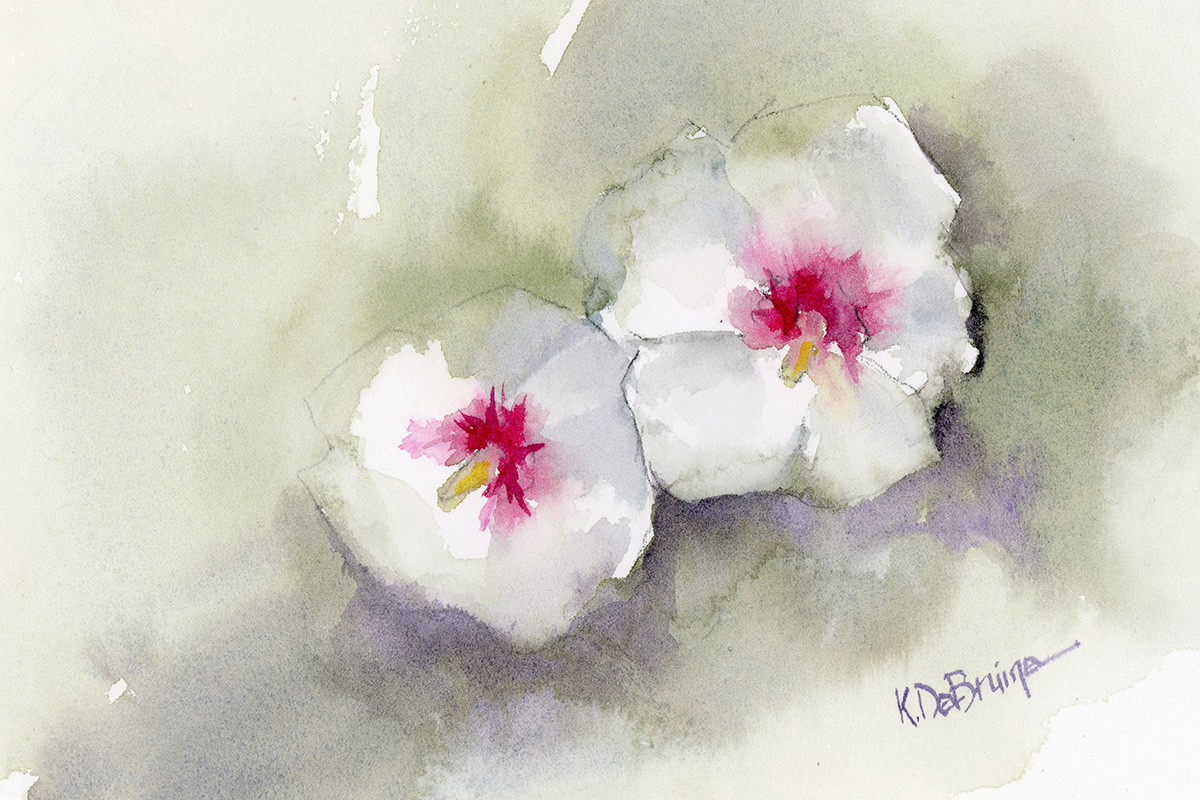The painting is a close-up, detailed watercolor portrait of two white flower petals with varying color accents. The larger flower is on the right, and the smaller one is on the left, placed centrally in a rectangular format. Each petal is outlined with a thin black line and features white with gray accents. The flower centers are rich with a blend of colors: the inner core is a vibrant mix of dark pink and light pink, merging into red with pink splotches, and a hint of yellow at the very center.

The background is nuanced, seamlessly transitioning from beige at the top, which appears to bleed into the flowers giving them a floating effect, to purple accents at the bottom of the petals that enhance the shadows. Surrounding the flowers, the background further fades from a dark gray to a lighter gray, eventually blending into white, creating a soothing visual gradient. Notably, there is an area in the lower right-hand corner that is completely white, devoid of any coloration, adding to the painting's ethereal quality.

Above the flowers are two distinct white splotches, suggestive of a soft overlay or design element. The artist's signature, "K.D. E.B.R.U.I.N.E" in cursive, is clearly visible at the bottom of the painting, adding a personalized touch. This elegantly composed painting showcases the artist’s skillful use of watercolor to blend and bleed colors together, creating an atmospheric and float-like effect around the distinct, softly shadowed flower petals.